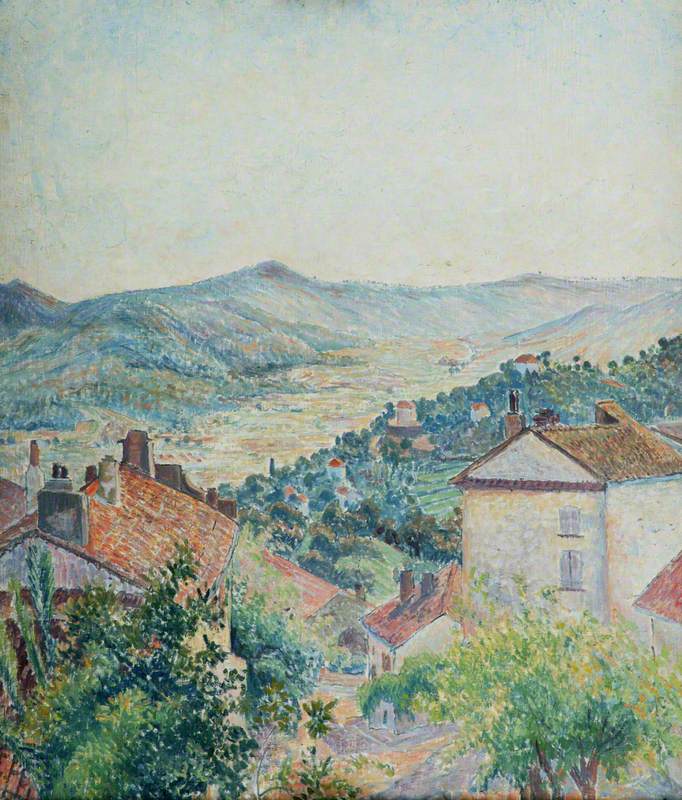This vibrant, impressionistic painting showcases a vast, far-ranging landscape from the vantage point atop a hill. The foreground is lush with trees in varying shades of green, while below, a charming village unfolds with numerous rooftops adorned with orange or brown shingles, and an array of distinctive chimneys. The style is pointillist, characterized by the artist's use of tiny dots and strokes of color that coalesce into a vivid and pleasing image. The mid-ground reveals additional buildings amidst verdant greenery, extending into a sprawling valley dotted with colorful structures that stretch out for miles. In the distance, blue skies meet the majestic outline of mountain ranges, adding depth and a sense of tranquility to the scene. The combination of hilly terrain, scattered rooftops, and vibrant pointillist technique provides a rich, immersive experience, drawing the viewer into the serene and picturesque setting.